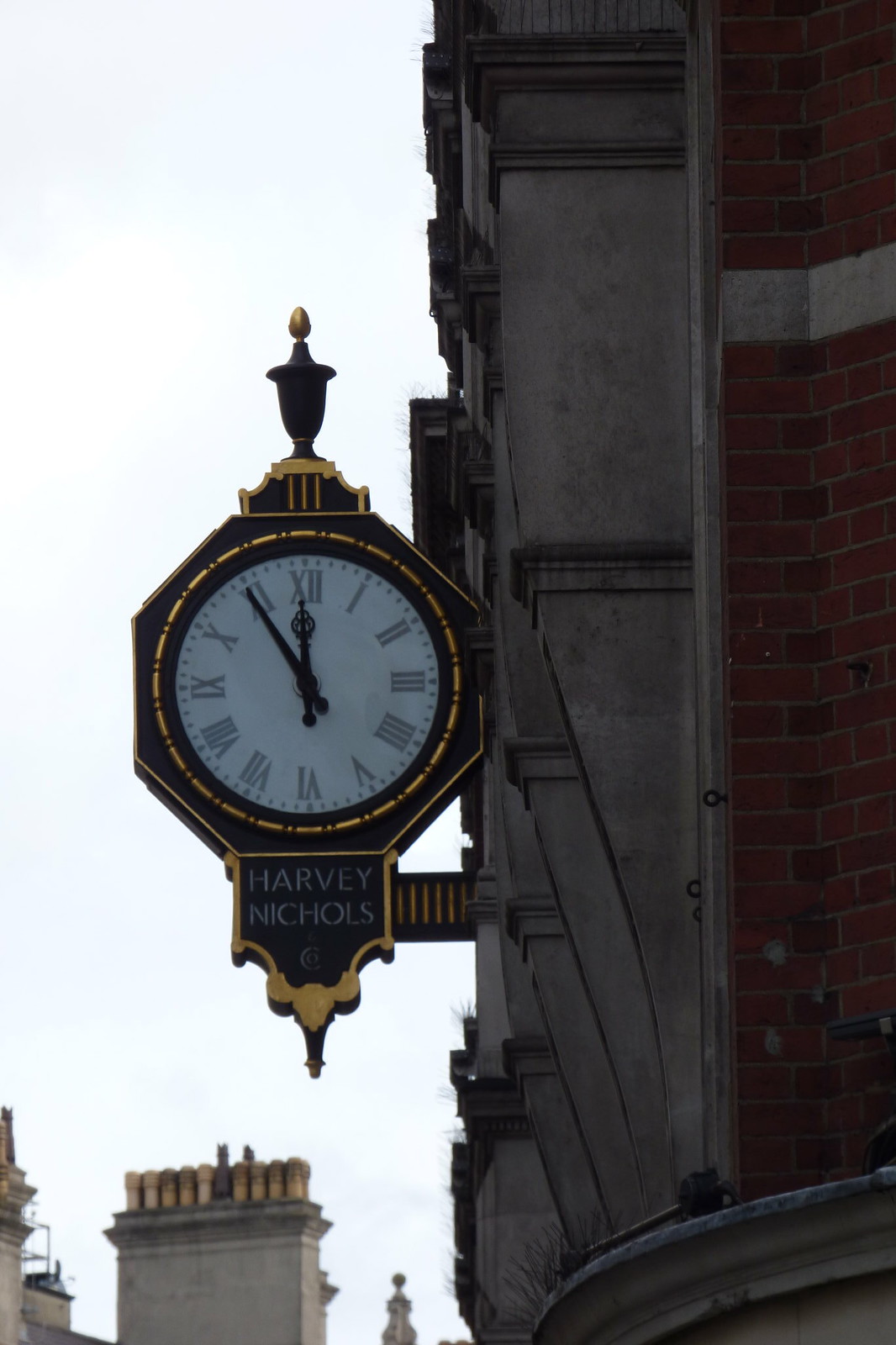The image depicts a vertically oriented, detailed photograph of an ornate clock jutting out from the side of a brick and concrete building. The six-sided clock, with an opulent black and gold border and a white face marked by Roman numerals, shows five minutes to twelve. Atop the clock, a dark metal vase-like ornament adds to its grandeur. The clock is mounted on a protruding metal arm, striped in black and gold, which extends from the building. Below the clock face, a black shield with gold borders contains the inscription "Harvey Nichols" in white capital letters. In the background, chimneys with various tubes emerge from another building, flanked by additional structures. To the right, a granite building topped with gold alongside an orange-red brick wall contribute to the rich architectural texture of the scene.